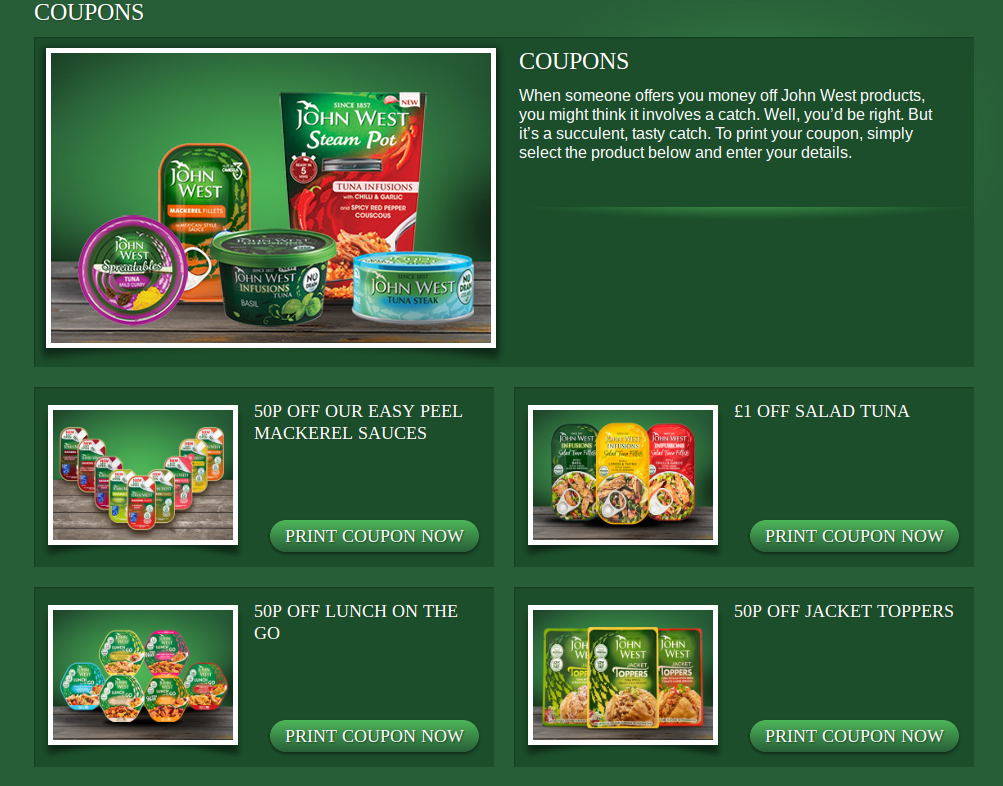The mock-up screen showcases the coupon section of what seems to be a grocery store's website, emphasizing deals on various John West products. The design features a medium-shaded green background with darker green rectangular panels. The top panel spans the full width of the section, with smaller panels arranged in a two-by-two grid pattern beneath it.

At the top left of the full-width panel, the word "Coupons" is prominently displayed in white. To the right, a message entices customers: "When someone offers you money off John West products, you might think it involves a catch. Well, you'd be right, but it's a succulent, tasty catch! To print your coupons, simply select the product below and enter your details."

Displayed below the message are various John West product images, including tuna steak, peas, and more tuna, packaged in a way that could be mistaken for cat food but are indeed human food offerings. A total of five product items are showcased with enticing offers:

- 50p off Easy Peel mackerel sauces
- £1 off tuna salad
- 50p off lunch on the go
- 50p off Jack toppers

Adjacent to each offer, "Print coupons now" buttons are provided for ease of access. The accompanying photos display three to ten packages per image, offering a visual idea of the available products.